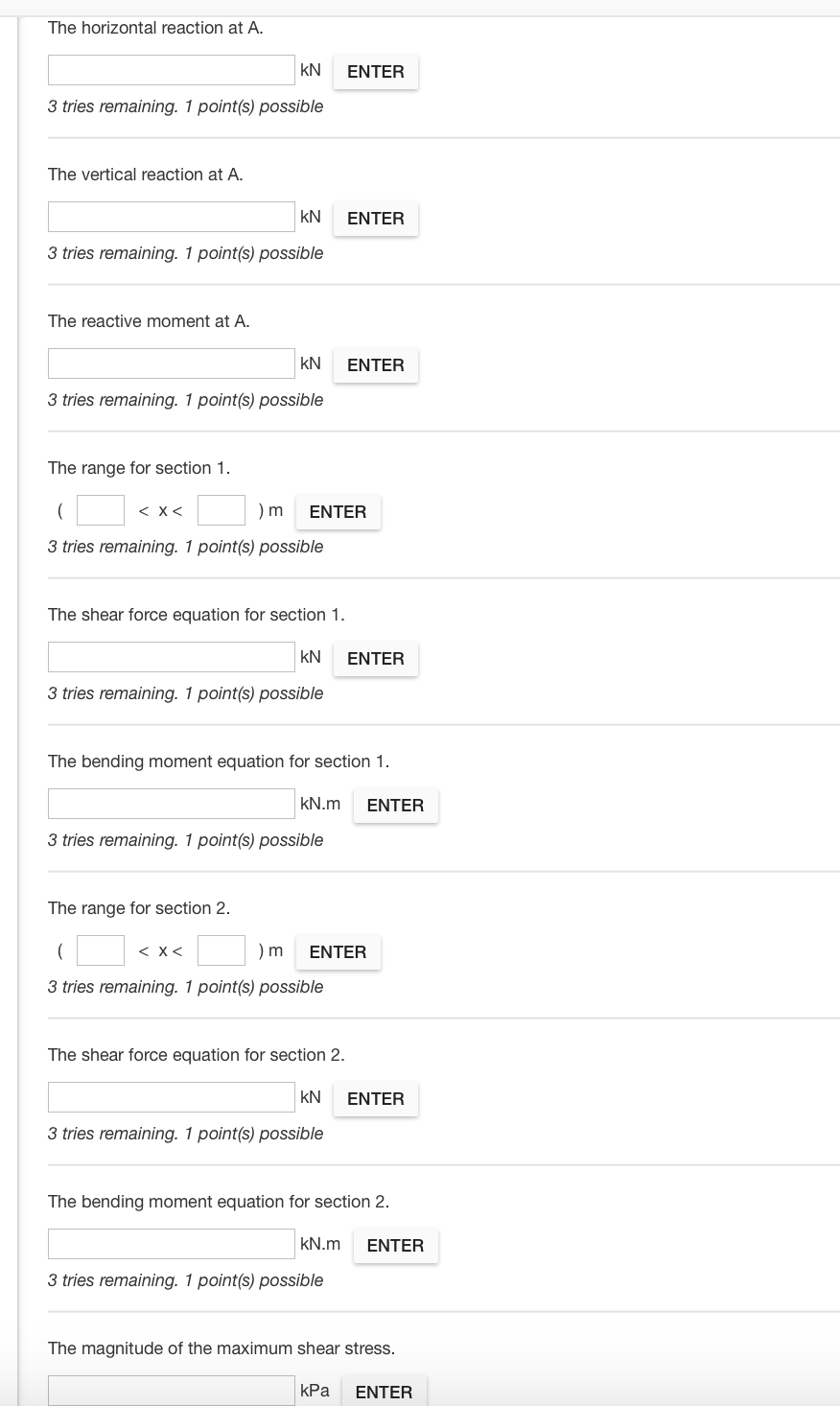This image depicts a structured list related to a problem-solving task, likely in the field of engineering or physics. At the top, it addresses "The horizontal reaction at A" with an associated text input box. To the right of this box, there's a label "K" for kilonewtons (KN), followed by an "Enter" button. Below this section, it indicates "Three tries remaining" and "One point possible."

The subsequent section is labeled "The vertical reaction at A," accompanied by another text input box, also labeled "K" for kilonewtons (KN), and an "Enter" button to the right.

Further down, it details "The reactive moment at A," providing a text input box with an "Enter" button next to it.

Following this, the list specifies "The range for section one," accompanied by a mathematical equation featuring text input boxes intended for numerical values.

Below this, the image delineates "The shear force equation for section one," succeeded by "The bending moment equation for section one."

Next, it introduces "The range for section two," then moves on to elucidate "The shear force equation for section two," and beneath that, "The bending moment equation for section two."

Finally, the list concludes with "The magnitude of the maximum shear stress," signaling the last entry in this informative and meticulous enumeration.